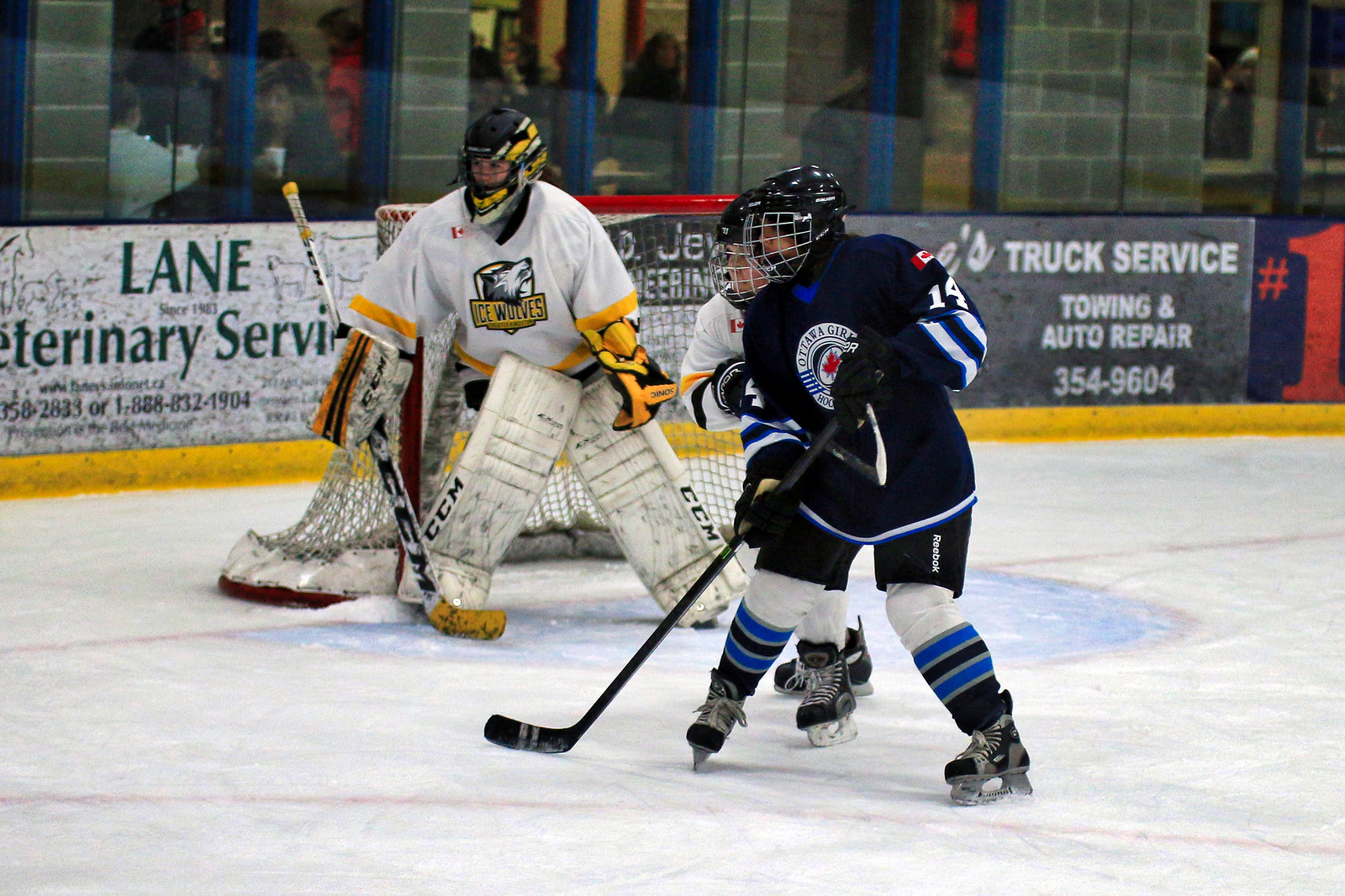In this dynamic ice hockey scene, three players take center stage on a large rink. The central player, wearing a black uniform accented with dark blue and white, notably sports blue and black striped socks and black shorts marked with a Reebok logo. Their jersey features the inscription "Ottawa Girls." Directly behind this player is a defender in a white jersey adorned with black and yellow accents. Further back, guarding the net, is the goalie from the Ice Wolves, easily identified by their black helmet and white jersey detailed with yellow accents and the team name emblazoned on the front. The rink is bordered by protective glass at the bottom of which various advertisements are displayed, including those for a lane veterinary service and another for truck service, towing, and auto repair, complete with a phone number. The backdrop reveals gray brick walls and spectators eagerly watching the game.